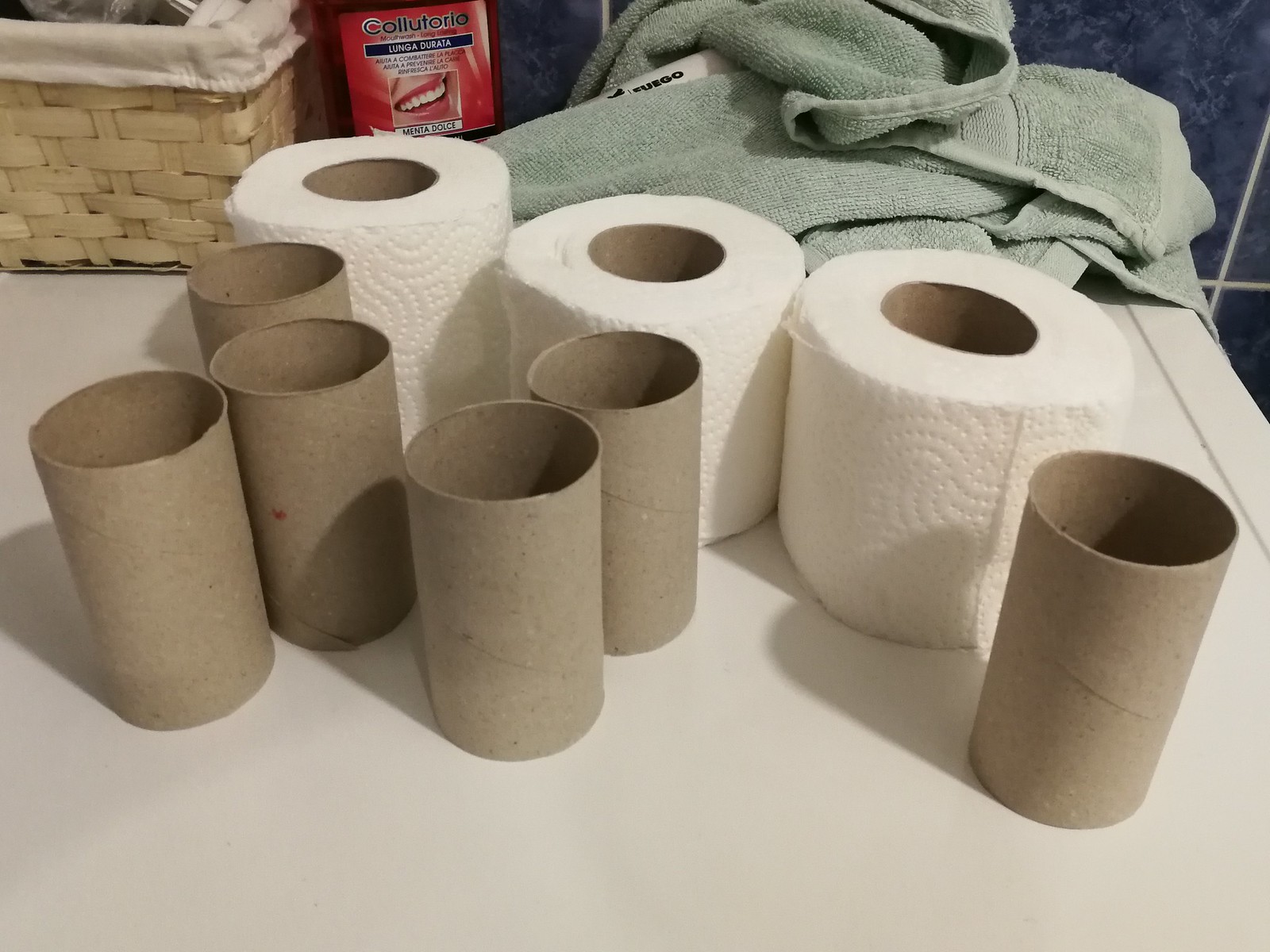The photo was taken indoors and features a white table with a light green, balled-up towel resting on its edge. On the table, three full rolls of white toilet paper stand upright alongside six empty brown cardboard tubes, arranged with five in a cluster and one off to the side. The dark blue tiled wall in the background has white grout lines. In the upper left corner, there's a light oak, handwoven basket with fabric draped over its edges, and next to it is an orange box labeled "Colutorio Lunga Durata," featuring a picture of a smiling woman's mouth with white teeth. A light source from behind the camera casts shadows of the toilet paper rolls onto the table's smooth surface.